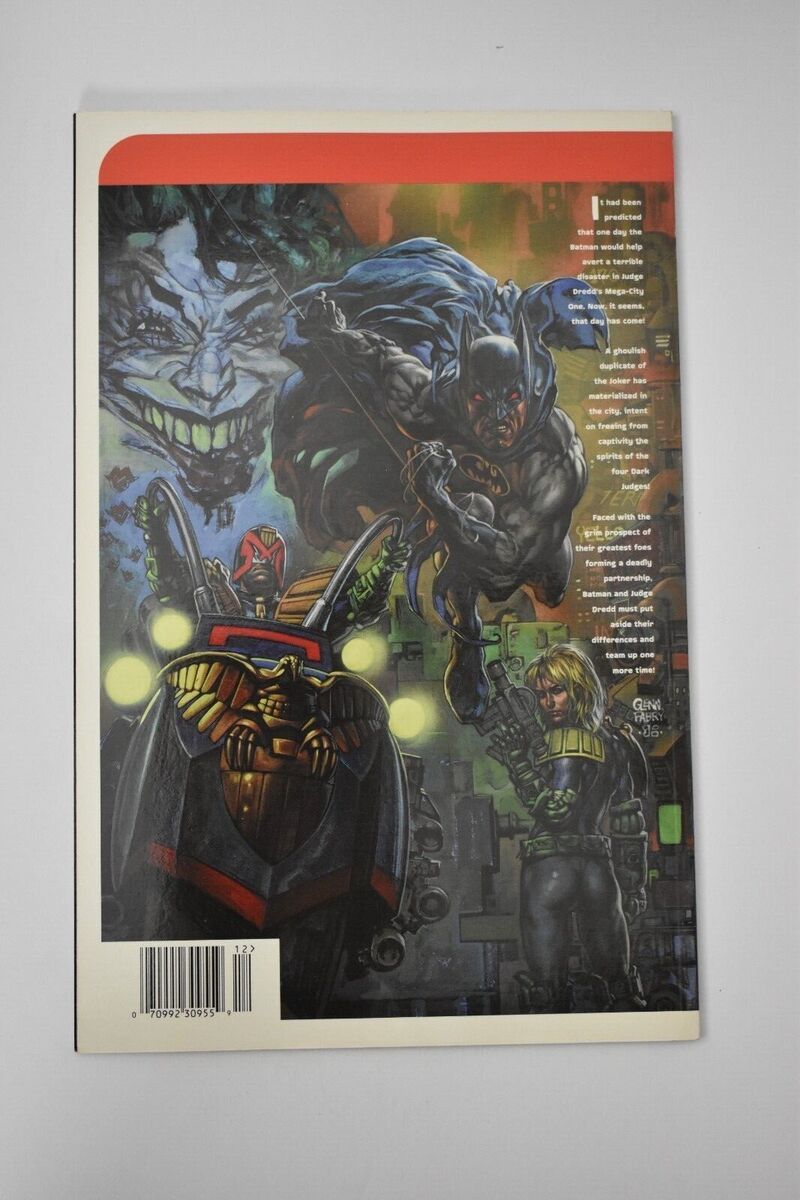The image is a scan of what appears to be the back cover of a Batman-themed graphic novel or comic book. The cover is vividly colorful and depicted in a rectangular portrait orientation, lying on a gray surface with noticeable shadows. Dominating the center is Batman, in his iconic black suit with a bat emblem and a blue cape, fiercely leaping or flying towards the viewer, his muscles prominently flexed and his red eyes adding an ominous touch.

The upper left features the Joker's face, characterized by green hair, stark white skin, and a sinister grin, which is slightly out of scale with the rest of the illustration. Below Batman to the right, a woman with bright yellow hair and dressed in a tight, metallic outfit with gold details is turning towards the viewer, holding a gun at her waist. Her back, clad in what looks like armor, is mostly visible.

In the lower left, a masked figure appears, riding a motorcycle or scooter that sports a golden eagle or falcon ornament at its front, suggesting a villainous presence. Across the right side of the cover, white text is presented in three small paragraphs against the vibrant background. The top of the cover is red, and a barcode is positioned at the bottom left corner. The entire cover exudes a dark, graphic novel style rather than a light-hearted cartoonish one. No visible price tag is present, emphasizing the detailed and elaborate artwork typical of a serious Batman narrative.